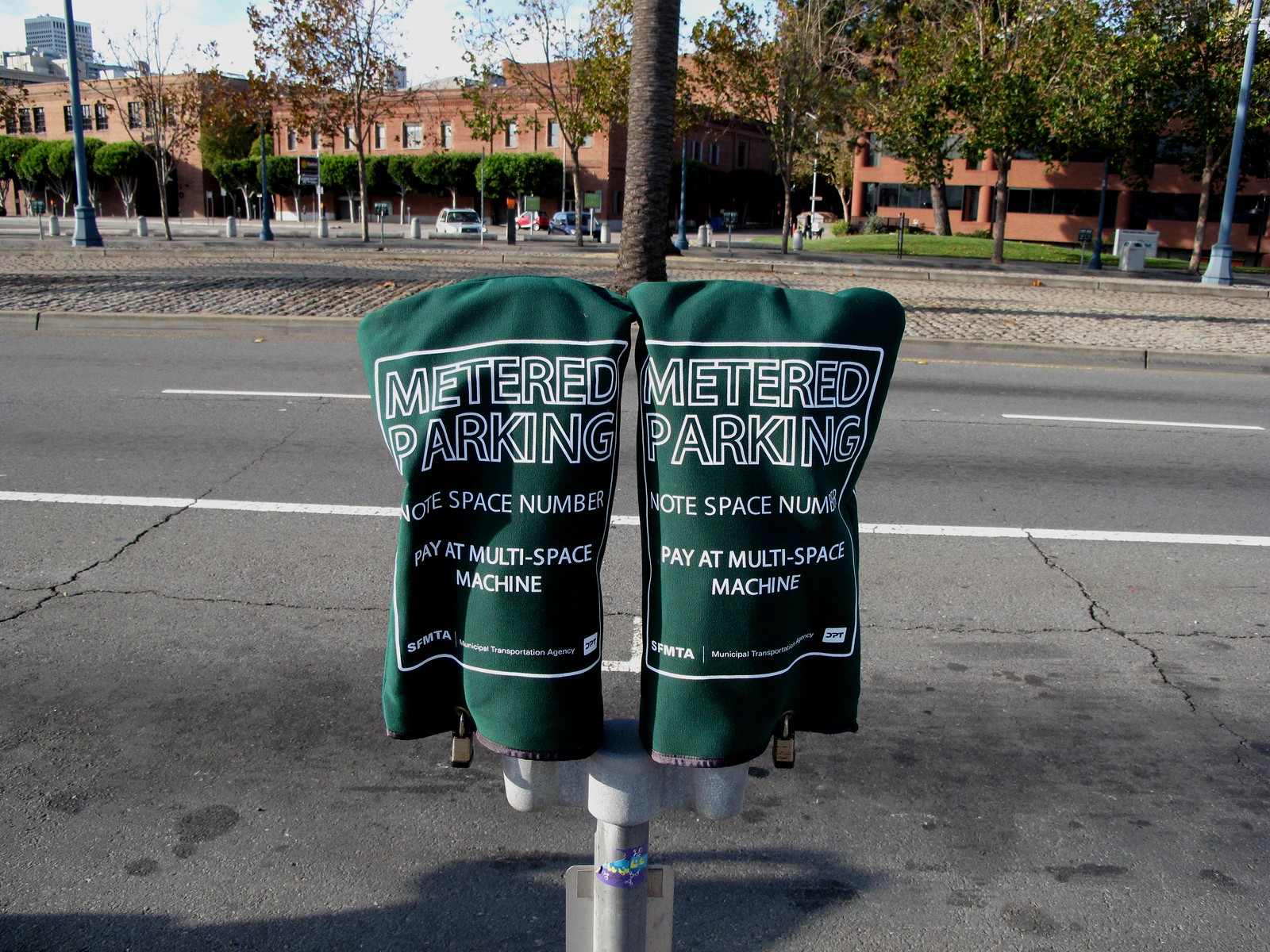The image vividly captures an outdoor urban scene centered on two traditional coin-operated parking meters, now out of use. These meters are thoroughly covered with green cloth bags, which prominently display the message: "METERED PARKING, NOTE SPACE NUMBER, PAY AT MULTI-SPACE MACHINE, SFMTA." Secured at the base with padlocks, these covers indicate a shift to a modern payment system likely accommodating credit cards and app payments. 

Positioned on a silver pole, the meters stand on a paved asphalt street marked by white lines and oil stains. Across this multi-lane road lies a varied landscape. Prominent in the middle background is a massive tree trunk with dark, thick bark, rooted in a cobbled median. Surrounding the area is a mixture of mature and youthful trees, their green leaves providing a lush contrast to a few brown-leaved specimens.

Beyond this natural scenery, a large, red-brick building—possibly a business complex or an institutional structure—stands surrounded by well-kept green grass. Scattered street lighting and parked cars populate the adjacent parking lot, creating a bustling urban tapestry. This detailed imagery highlights the transition from old to new in the city's parking infrastructure amid a lively and diverse streetscape.